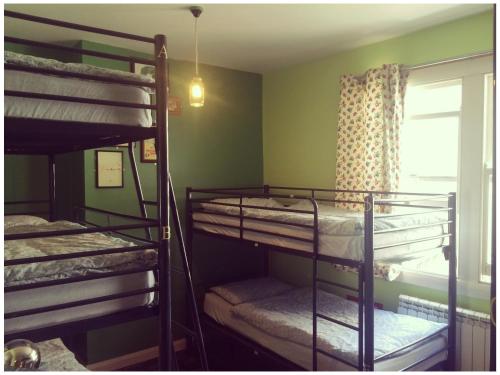The image, slightly wider than it is tall, depicts a room with olive green and light green walls, where they meet in approximately the middle. The ceiling is white, and on the right-hand wall, sunlight streams through a partially open window with white framing and a cream-colored curtain adorned with indistinct green and rose-colored spots, pushed to the side, forming folds. The dark floor has white baseboard trim around the perimeter.

In the left third of the image, there is a towering bunk bed that reaches nearly to the ceiling, apparently three-tiered. These beds, featuring plain brown metal railings, host white mattresses with fitted sheets and some folded bedding in muted greens, browns, and whites. A brass ball is visible in the lower-left corner. The taller bunk bed is juxtaposed by a smaller, double-tiered bunk bed positioned towards the center-right corner of the room, extending along the light green wall to the midpoint of the window. This smaller bunk is built from similar brown metal and supports white mattresses, with a more accessible built-in ladder that contrasts with the leaning ladder of the taller bunk.

The room features additional details: a few framed pictures hanging on the dark green wall and a heating unit near the window. Centered in the room is a tubular glass light fixture, hanging down about two feet on a plain white stem, illuminating the room with faint beams radiating from its clear glass jar-like shade.

Together, these elements construct a detailed, multi-layered depiction of a brightly lit, somewhat utilitarian room, possibly in a dormitory or barracks, designed with practicality in mind for both children and adults.